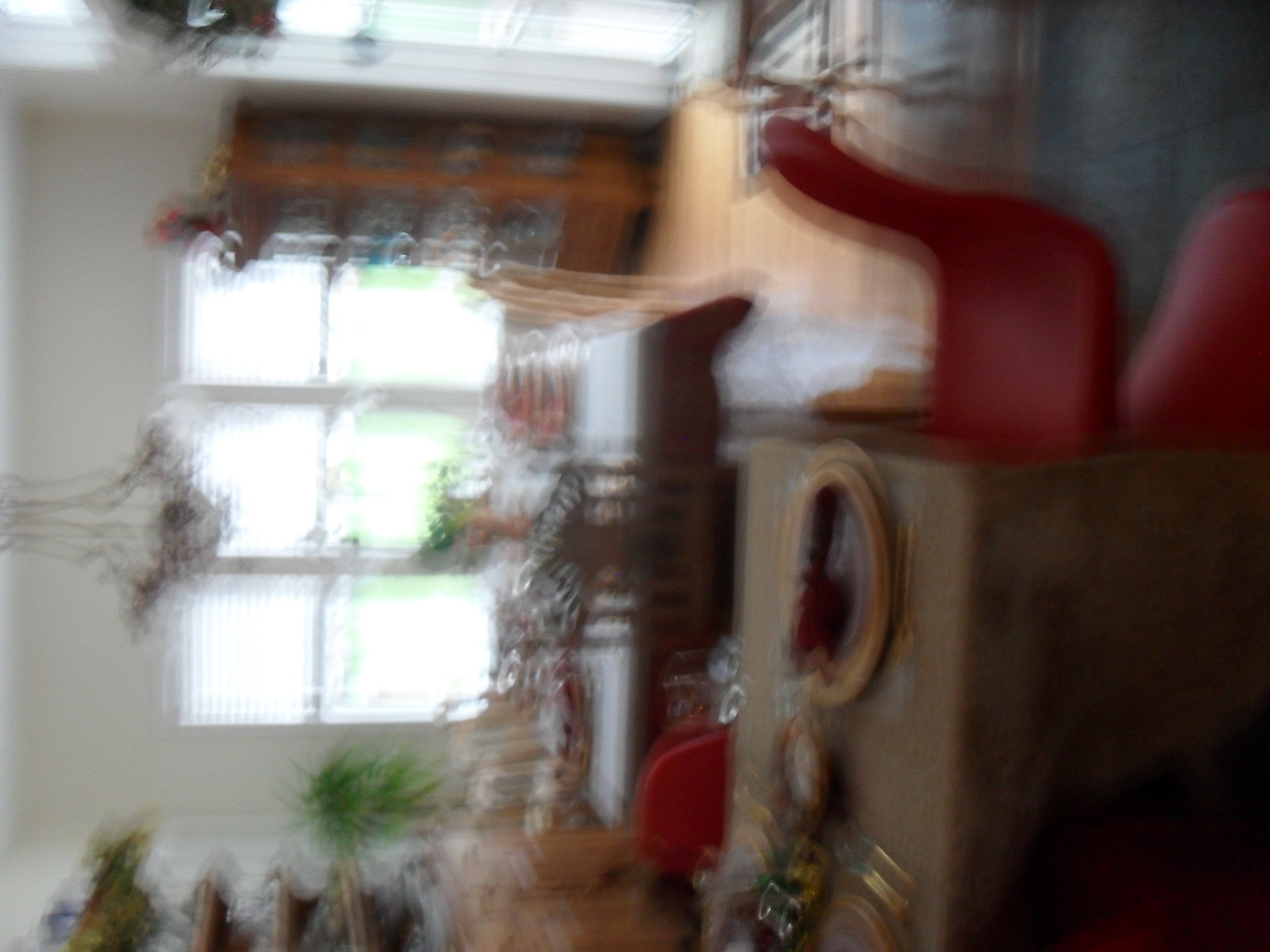The image depicts a dining room with an ornate and cluttered interior, presented at a tilted angle. The room is bathed in daylight streaming through three two-paneled windows in the background. A chandelier hangs from the ceiling over a central table adorned with a flower bouquet. The table features a tan tablecloth, gold silverware, and a dish. A red plastic chair is positioned at a smaller, separate table in the foreground, which appears to be set for a child.

To the right, against a wooden wall, are multiple cabinets filled with glassware and various items, including a distinctive box with a notable yellow circle and glass front, accompanied by similar shapes below and surrounded by intricate gold lines. These cabinets also feature plants and other decorations on top. The room has hardwood floors with an area rug near a sliding door, allowing more light to flood in. The overall image is very blurry and out of focus, emphasizing the bright, cluttered, and ornate nature of the space.